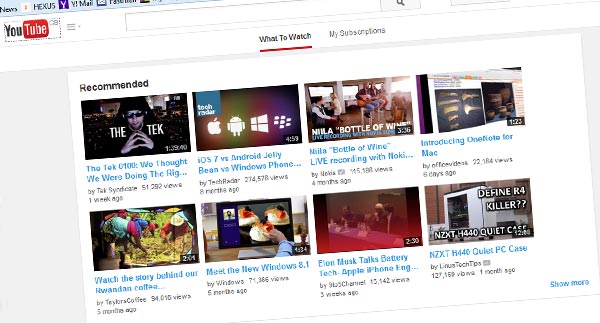The image depicts a slightly twisted YouTube interface, appearing tilted to the left. At the top, prominently in red, is the YouTube logo with a search button to its right. Below the logo, a bolded "What to Watch" section is underlined in red, and the currently displayed category is "Recommended Videos."

The main section features two rows of video thumbnails, with four thumbnails per row. Each thumbnail provides a snapshot of its respective video, including the title, channel name, view count, and how long ago it was uploaded. 

The first video thumbnail in the top row is titled "The Tech 0100: We Thought We Were Doing the Right..." and was uploaded one week ago. Next to it is "OS7 vs. Android Jelly Bean," followed by a music video live recording, and then "Introducing OneNote for Mac."

The second row starts with a thumbnail titled "Watch the Story Behind Our Rwanda Coffee," showcasing a group of people picking coffee beans in a field. Alongside it is "Meet the New Windows 8.1," featuring someone working on a laptop. Further to the right is "Elon Musk Talks Batteries," and "NZXT H440: A Quiet PC Case."

In the bottom right corner of the interface, there is a blue button labeled "Show More," inviting users to browse additional videos.